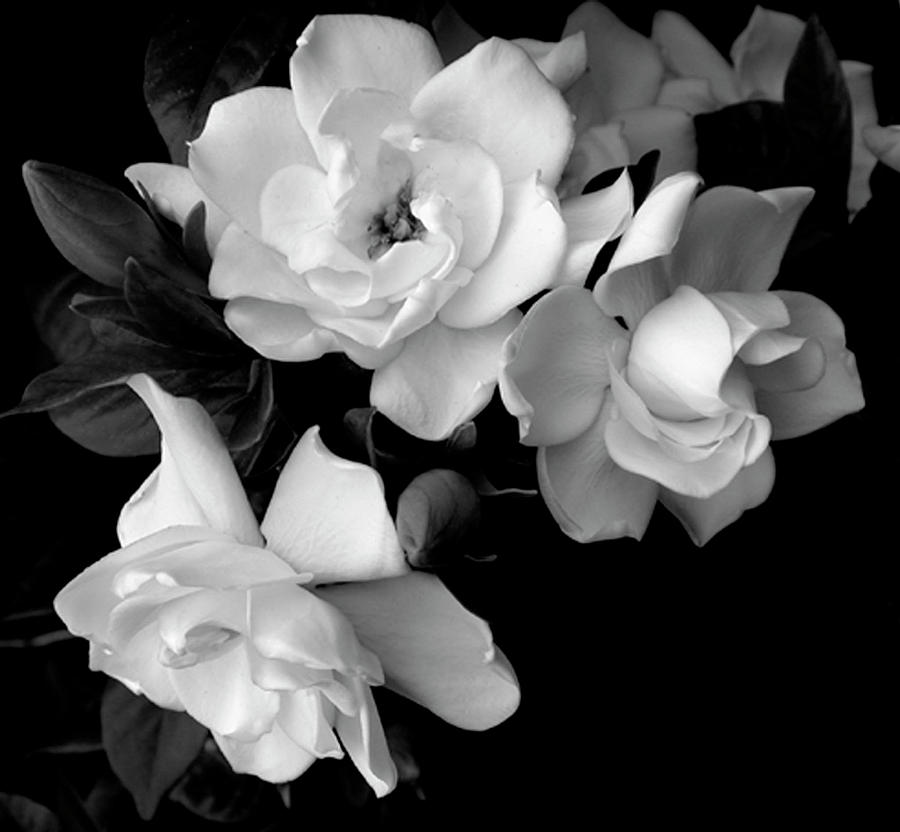This black and white photograph features a striking and minimalist composition of white flowers set against a dark background. The flowers, which appear to be either gardenias or magnolias, have large, open blooms that dominate the frame. There are four open flowers arranged prominently, with the petals blown out to pure white, making them stand out vibrantly against the contrasting black background. In the upper left corner, a single bud is visible, yet to bloom. The dark foliage behind the flowers adds depth and contrast, further emphasizing the purity and brightness of the white petals. The overall effect is both somber and artistic, with the luminous flowers evoking a sense of melancholic beauty.